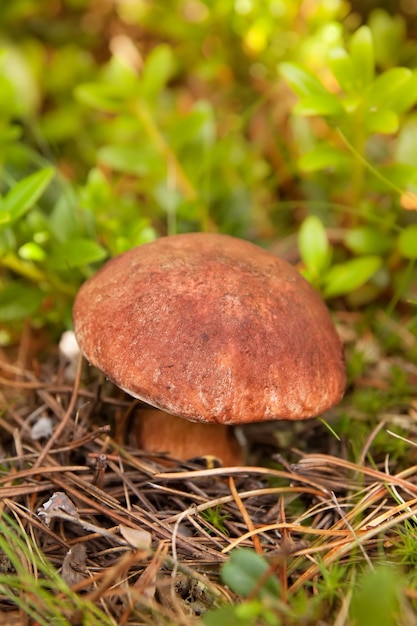This nature photograph captures a prominent brown mushroom with a large, wide cap and a stout stem growing from the forest floor. The mushroom, tinged with hints of red, stands out prominently in the center of the image. It's surrounded by rotting foliage, an array of brown branches, and scattered pine needles, which enhance the earthy environment. The background, slightly blurred to emphasize the mushroom, reveals bright green leaves and hints of flora basking in dappled sunlight. The scene, bathed in natural daylight, provides a tranquil glimpse into a rich, forested habitat with low-lying shrubs and varied greenery. The portrait orientation of the image accentuates the upward growth of the mushroom.